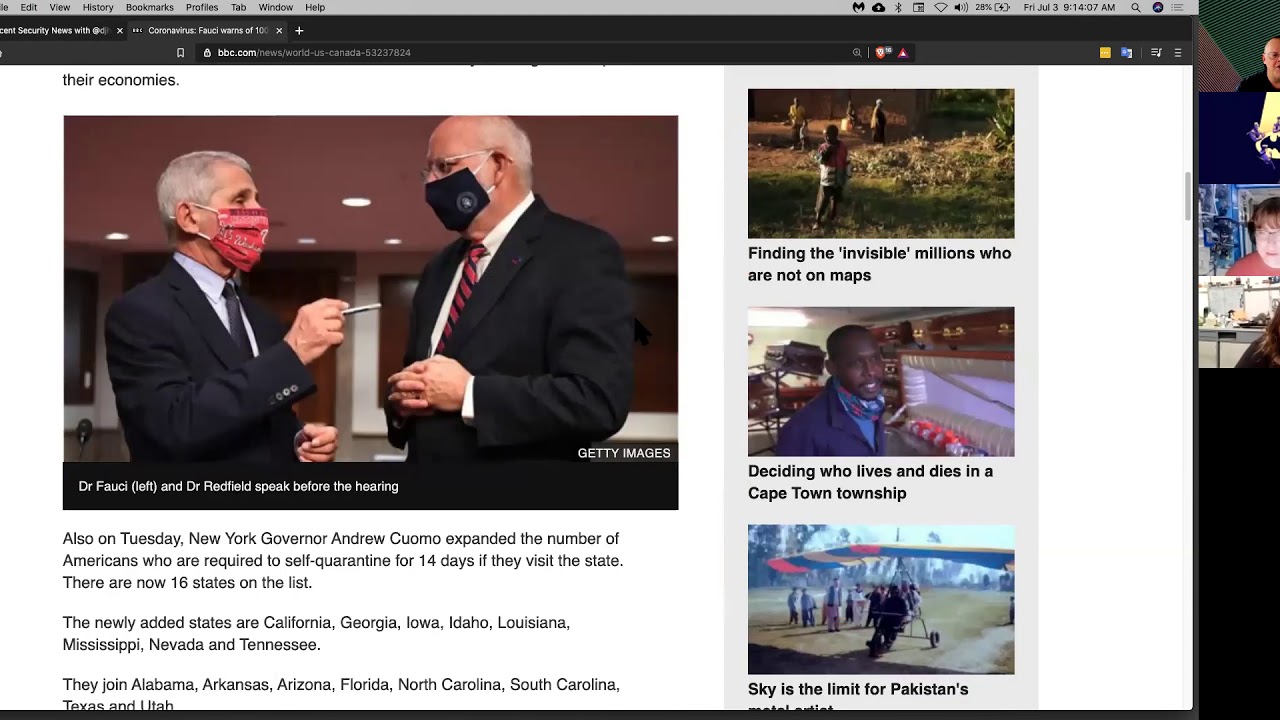A screenshot captured from a desktop computer displays the homepage of the website bbc.com. The upper portion of the image features the browser’s gray status bar along with two additional gray navigation bars situated below it. The web address “bbc.com” is clearly visible on the second gray bar. 

Dominating the left side of the screen is a large, prominent image showing two men dressed in suits. The man on the left is adorned with a red face mask and holds a gray pen directed toward the man on the right, who is wearing a green face mask. To the right of this large image, three smaller, colorful images are aligned vertically. Directly below the topmost of these smaller images, a black text caption reads, "Finding the invisible millions who are not on maps."